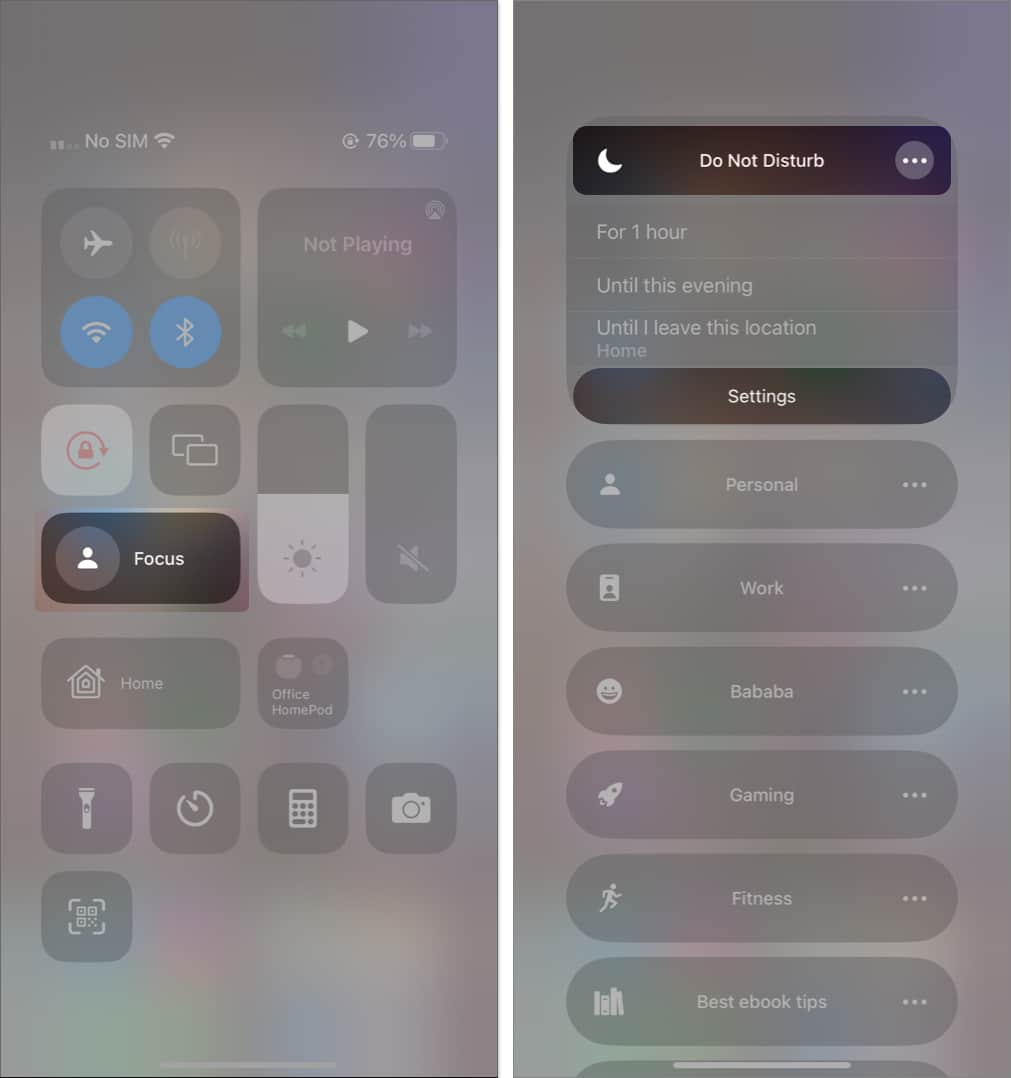The image features a split screen with both sides displaying a muted gray background that gives an overcast ambiance. On the left side, there's a screenshot from a cell phone showcasing various notification icons and settings. At the top, the text "NO SIM" is prominently displayed in capital letters, indicating the absence of a SIM card. Towards the left corner, the battery level is shown at 76%. Below the text, a series of icons are arranged vertically: first, a small airplane icon symbolizing Airplane Mode, followed by a blue circle with stylistic lines presumably indicating some connectivity feature, and another blue circle without any inner design.

To the right of these icons, there's a square marked "Not Playing," denoting no current media playback. Within this square are controls featuring two arrows pointing left, two arrows pointing right, and a bold white arrow in the center, likely representing media navigation buttons. Further down, there's a small white square containing a red lock icon encircled, alongside two rectangles within a gray square, possibly indicating security features or apps.

Directly below is a long rectangular area indicating the brightness level of the screen, positioned at the midway point. To the left of this bar, within a black rectangle, the word "Focus" is displayed accompanied by a central circle icon, suggesting a focus mode. On the right edge, a small crescent moon icon appears, located in the upper corner, signifying the "Do Not Disturb" mode. Beside this, the text "Do Not Disturb" is inscribed next to a circle featuring three horizontally aligned dots. A couple of inches below, within another black circle, the word "Settings" is visible.

The right side of the image is not as clearly detailed, which maintains the uniform gray tone, thereby emphasizing the detailed intricacies shown on the left side of this composite image.